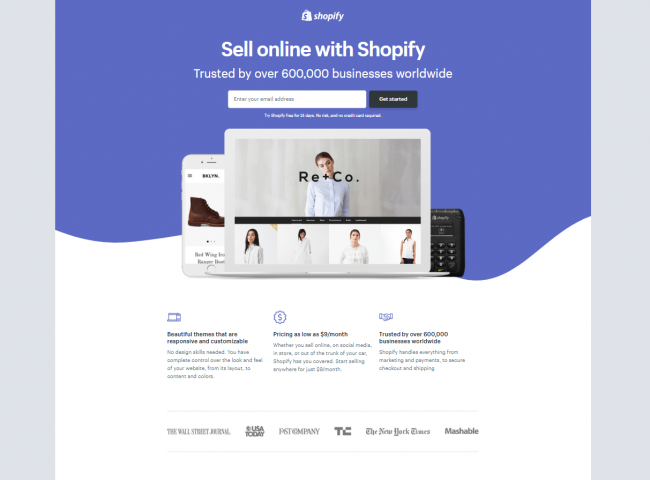The screen capture appears to be an advertisement, flanked by thin gray bars on either side. The ad features a blend of purple and white backgrounds with several key components. At the very top, in white text, is the Shopify logo, accompanied by a small shopping bag icon with a dollar sign. The headline reads, "Sell Online with Shopify," followed by a subheading that states the platform is "Trusted by over 600,000 businesses worldwide."

Beneath the headline is a white search box and a prominent black "Get Started" button, with a brief promotional sentence in white text underneath. The ad also includes images of various devices: a white cell phone displaying brown boots with black text, a white laptop showing simulated website images with a model dressed in white labeled as "RE + CO," and a black device with buttons on it.

Further down, there are three purple icons depicting a laptop, a circle with a dollar sign, and two cartoon hands shaking, each accompanied by a paragraph of text in black font. Below these icons, the names of notable companies—The Wall Street Journal, USA Today, PST Company, TC, The New York Times, and Mashable—are listed, separated by a thin gray bar above and below.

While the font in the advertisement is somewhat challenging to read, the overall layout is clear and informative, effectively communicating the benefits of using Shopify for online sales.